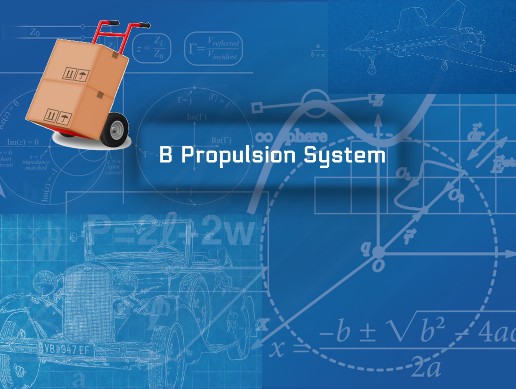This image appears to be a highly detailed engineering or physics design poster with a predominant blue background featuring various shades - darker blue in the upper right-hand corner, lighter blue in the bottom left corner, and medium blue in other sections. The central focus of the poster is a blue rectangle with the white text "B Propulsion System." In the upper left-hand corner, there is a red dolly carrying two brown boxes. Scattered throughout the background are numerous mathematical equations, diagrams, and symbols, including an outline of a jet airplane in the darker blue section and an old T-model vehicle in the lighter blue section. The intricate overlay of designs and calculations adds depth and complexity to the image.